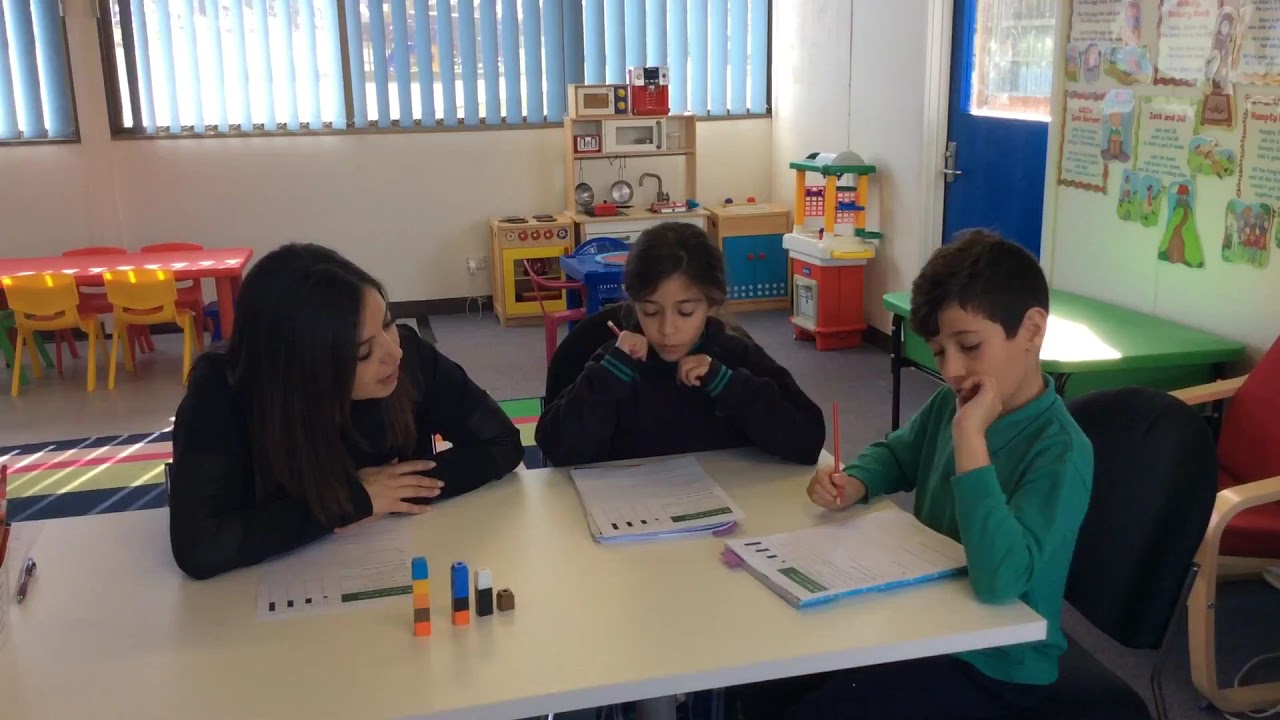In this detailed image set within a lively school room, likely a preschool or early elementary classroom, we see a teacher engaging with two young students. The classroom is filled with child-sized furnishings, including small tables and chairs, a miniature kitchen playset, and vibrant decorations. Prominently, there is one adult-sized chair at the table. The teacher, with black hair and wearing a long-sleeve black shirt, is positioned to the left, holding a paper. 

Two children, approximately around the age of 10, are seated beside her. The young girl, in a black jacket and holding a pencil, focuses intently on her worksheet, while to her left, a boy in a teal sweater also attends to his workbook. The scene includes several engaging elements: multi-colored Legos are scattered on the table, and the room is bathed in natural light streaming through shades. In the background, a blue door with a window halfway up stands out, accompanied by colorful red and yellow chairs and green and red tables. Various toys and educational materials are displayed around the room, with posters and learning resources adding to the vibrant, nurturing learning environment.